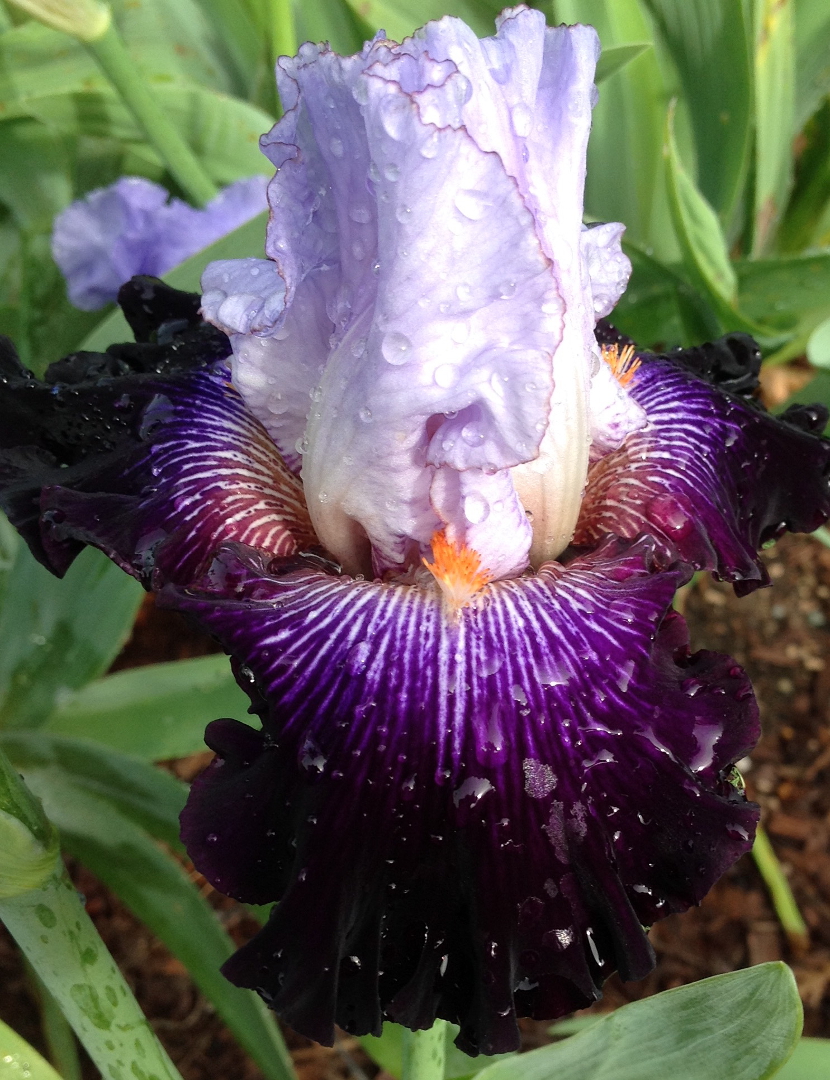A stunning close-up of a partially open purple flower, featuring a dark, mesh-like base from which intricate details emerge. Three prominent, cup-like petals, elegantly striped in purple and white, reach upwards. In the center, a small cluster of vibrant orange structures stands out. The flower's pinnacle showcases a tightly-knit clump of white, dewy petals, glistening with moisture and not yet fully unfurled. The background fades into a serene blur, revealing additional hints of a purple flower and a lush array of green leaves and stems, providing a rich, natural backdrop to this exquisite bloom.